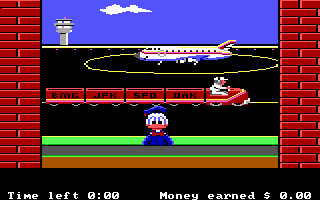The image is a detailed screenshot of an old vintage 2D pixelated game. The screen capture appears to have been taken from a small, rectangular horizontal monitor, reminiscent of an arcade display. The image has no external borders but features a black bar at the bottom. On the left side of this bar, white text reads "Time Left: 0.00," and on the far right, the text "Money Earned: $0.00" is displayed.

The main scene above the black bar depicts an airport setting. Central to this image is a pixelated duck, positioned prominently in the middle of the frame. In the background, a runway extends into the distance. Alongside the runway, a vehicle is seen driving, likely a luggage transport cart. Situated on the runway's black asphalt is an airplane, encircled by a yellow outline. The runway is flanked by two brick walls, focusing the viewer's attention on the central scene. The upper part of the image showcases a blue sky with a single white cloud situated to the right. To the left of this cloud, a control tower can be seen in the distance, completing the airport's landscape.